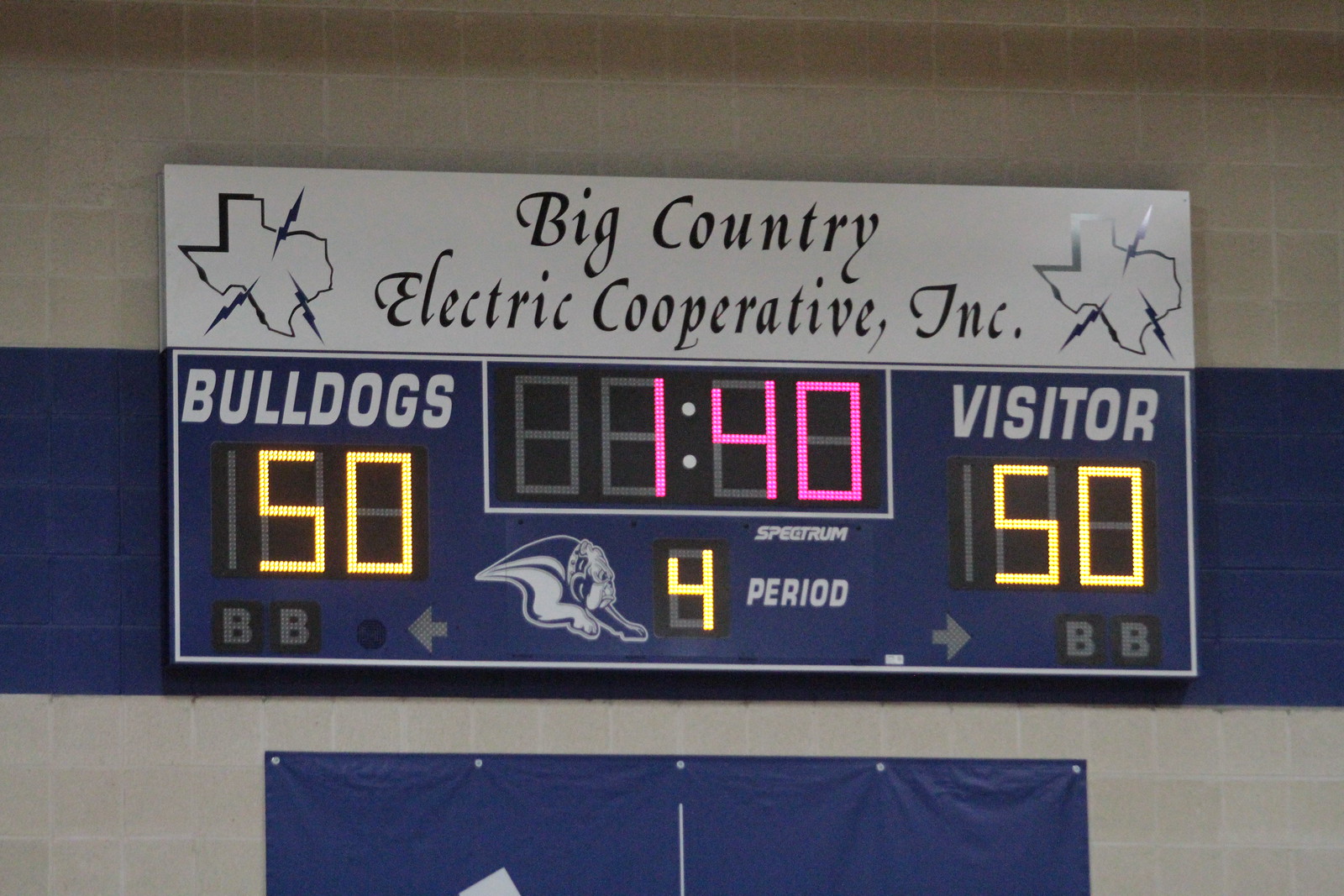The image depicts a prominently displayed, bolted scoreboard against a gray concrete block wall, divided by a blue strip. At the top of the scoreboard is a white rectangular panel featuring black line drawings of the state of Texas on both sides, each emitting three lightning bolts. In the center, bold letters read "Big Country Electric Cooperative Inc." Below this, the scoreboard itself has a blue background with white and gold text. On the left, "Bulldogs" is displayed with a score of 15 points, while on the right, "Visitor" also shows 15 points. Central to the display, pink LED numbers indicate the game time as 1 minute and 40 seconds, with "4" denoting the period positioned below. The score and time are in yellow and pink respectively. The overall color scheme combines blue, white, gray, and splashes of yellow and pink.